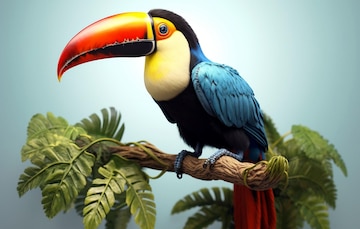This detailed illustration portrays a vibrant Macaw prominently featured in the center, resembling either a print or painting. The bird boasts a large, sharp beak, predominantly orange with black on the bottom. The area surrounding its eye is yellow, while the eye itself is blue. The Macaw's head and throat are black, transitioning to a vividly yellow chest. Its wings display a striking light sky blue. The bird's blue feet grasp a brown tree branch adorned with green leaves. The background of the image is a blend of grayish blue, with a brighter white spotlight directly behind the bird, enhancing its colorful plumage.